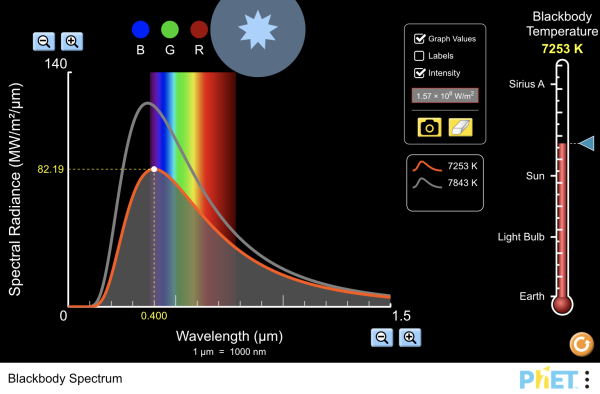The image is a detailed scientific diagram illustrating "Spectral Power Density as a Function of Wavelength." The background is black, providing contrast for the various colored elements. On the left side of the image, from top to bottom, "Spectral Power Density (W W/m²/µm)" is written in white. Adjacent to this text is a white vertical bar with indicators from zero at the bottom to 500 at the top, separated by two small blue clickable icons—one with a slashed magnifying glass and another with a positive magnifying glass. 

At the bottom of the image, the label "Black Body Spectrum" is prominently displayed. The graph itself consists of colored bars and a color spectrum rectangle placed as the background. In the top corner of the image, labeled "Black Body Temperature," is a large thermometer extending nearly the full height of the diagram. It is white with a pink center section and shows a temperature of 7,250 K. To the left of the thermometer, labels indicate "Sirius A," "Sun," "Light Bulb," and "Earth."

Just above the thermometer, the diagram features three colored dots (blue, green, and red) labeled "B," "G," and "R" respectively. Below these, a spectral power density graph is overlaid on the color spectrum rectangle, showing data lines in orange and gray. The graph indicates that spectral power is higher in the indigo and blue regions and less so in the reds. In a smaller rectangle underneath the main graph, the orange and gray lines are described, displaying their behavior across the graph.

Overall, the diagram provides a comprehensive visual representation of spectral power density related to different black body temperatures, complete with intricate labeling and color coding to enhance clarity and detail.